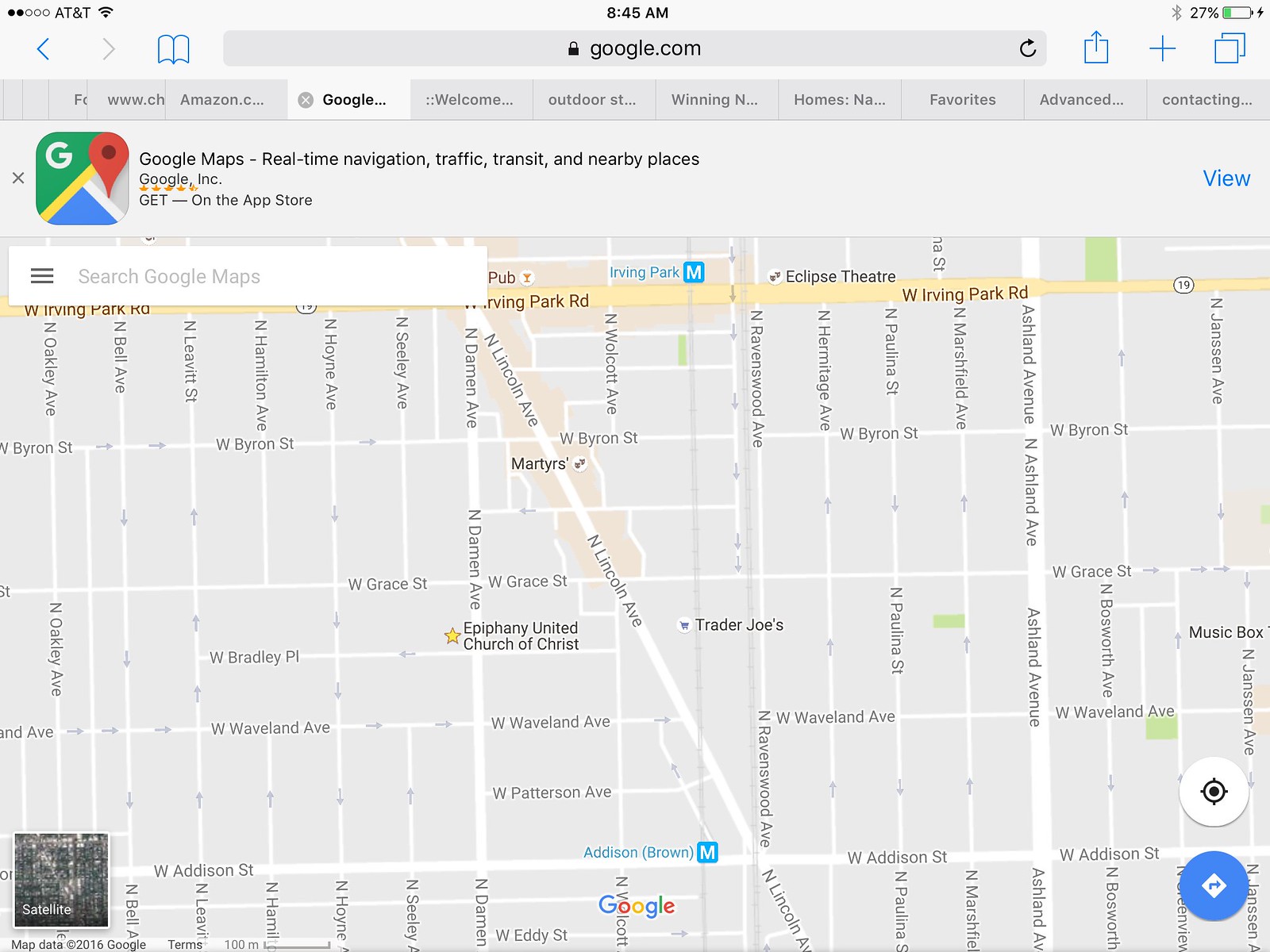This image captures the screen of a Google Maps interface displayed on a device, possibly a tablet, computer, or phone. The map prominently features a city's street layout, including several noted thoroughfares and locations. West Addison Street spans horizontally across the map, while Ashford Avenue runs vertically. North Lincoln Avenue is depicted with a diagonal vertical orientation, and North Damien Avenue runs vertically. Highway 19, also known as West Irvington Park Road, stretches horizontally. Key landmarks on the map include the Epiphany United Church of Christ situated on North Damien Avenue, Addison Brown located on West Addison Street, and the Eclipse Theater along West Irvington Park Road. Additionally, users can switch to satellite view via an option on the bottom left corner or access directional features using the button on the bottom right side of the map.